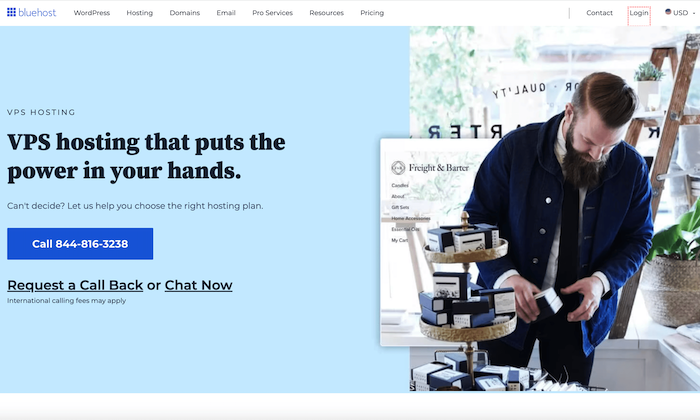Screenshot Description:
The image is a screenshot of the homepage of a website. At the top left corner, the title "Bluehost" is prominently displayed. Just below this, towards the middle-left of the image, the text "VPS Hosting" is visible. The main title, positioned near the center-left, reads, "VPS Hosting That Puts the Power in Your Hands." Below this main title, there is a prompt saying, "Can't decide? Let us help you choose the right hosting plan." Accompanying this prompt is a call-to-action button that says "Call 844-816-3238." Below this button, there are additional options: "Request a Call Back" and "Chat Now." In smaller text beneath these options, there is a disclaimer stating, "International calling fees may apply."